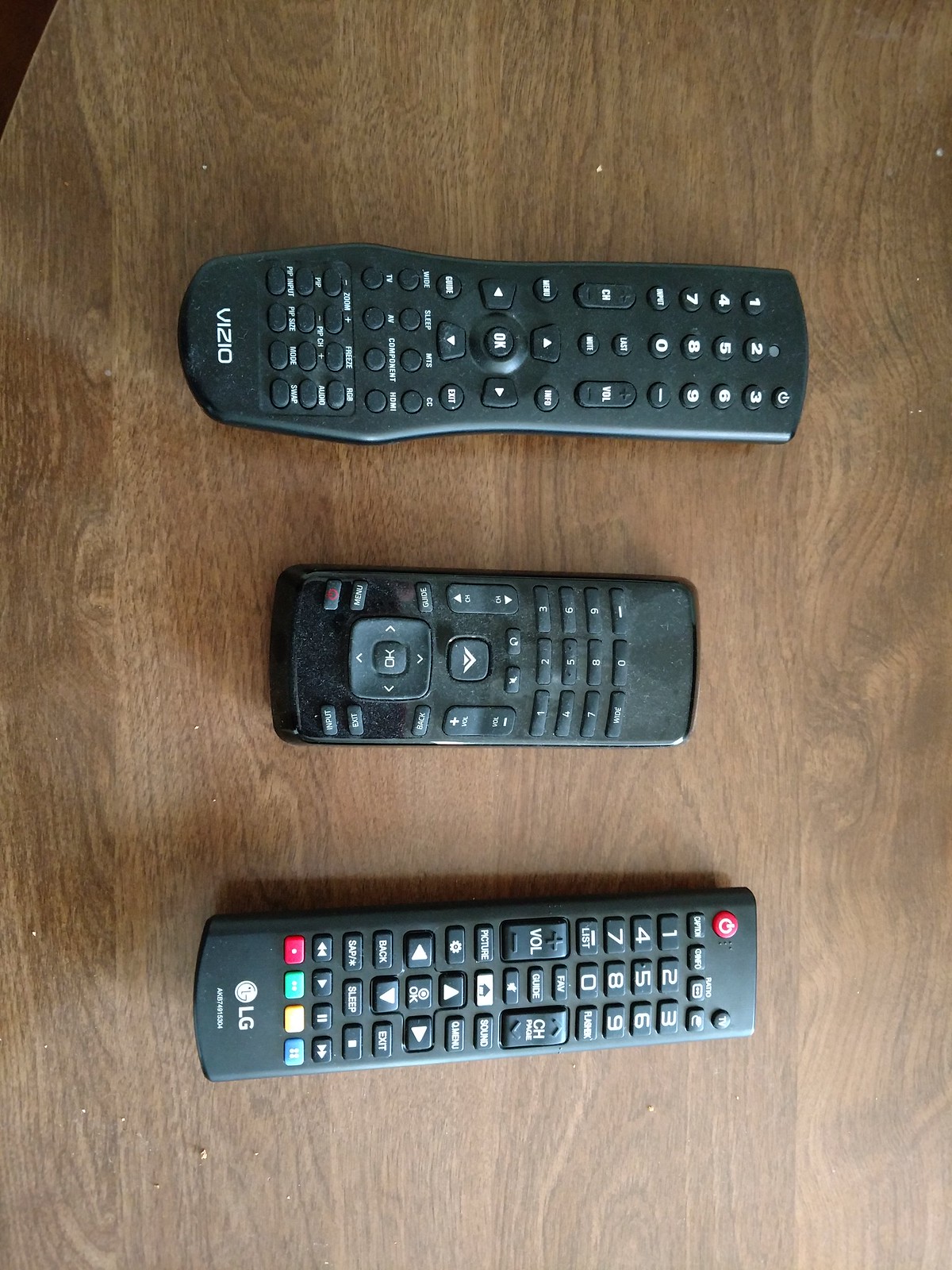The image showcases three different TV remote controls, neatly arranged horizontally on a flat, wooden table. The bottom remote, slightly larger and branded by LG, features a circular red power button at the top and four color-coded buttons—red, green, yellow, and blue—at the bottom. This remote is all black and includes a mix of numerical and functional buttons. The middle remote is the smallest, about 4 inches long, and lacks any branding. It's all black with black buttons that have white text and numbering, including a prominent "CH" button for channel changes and arrows for volume adjustments. The topmost remote belongs to Vizio, is slightly longer, and is distinct with its white Vizio logo at the bottom. It contains black buttons with white text, including numbers 0 through 9 and functional arrows. This one is oriented differently from the others, facing towards the right, and is also all black. All three remotes display a consistent design theme of black with white text, while resting on the brown surface of the table.